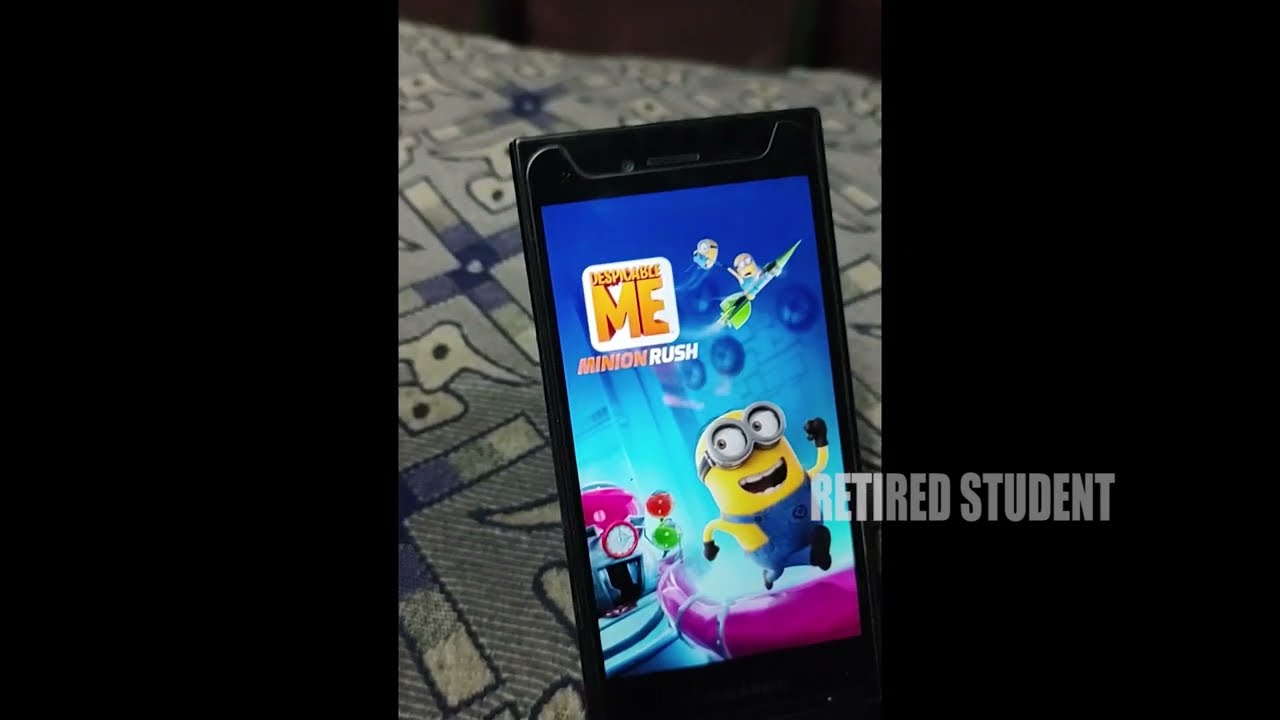In this image, we see the home screen of the mobile game "Despicable Me: Minion Rush" displayed on a rectangular, black smartphone. The screen prominently features the Despicable Me logo on the top left, with "Despicable" in small font and "Me" in a bright orange, large font, enclosed in a cube-like border. Below this, the game's title "Minion Rush" is written with "Minion" in dark orange and "Rush" in white. A yellow Minion character, recognizable from the Despicable Me movies by its goggles, is seen running on a purple pipe located at the bottom right of the game screen. In the background, to the left, there is a cartoonish house, and in the top right, two other Minion characters appear, one riding a green rocket and the other on a jetpack, flying above the Minion on the rocket.

The phone is being held up against what appears to be a bedsheet, draped in light gray with a pattern of crosses and skulls in the background. Written in gray text near the bottom right of the image, slightly overlapping the phone's screen, is the phrase "Retired Student." The image itself is framed by thick black borders on both the left and right sides, indicating the photo was likely cropped and angled in a specific way to capture this detailed scene.